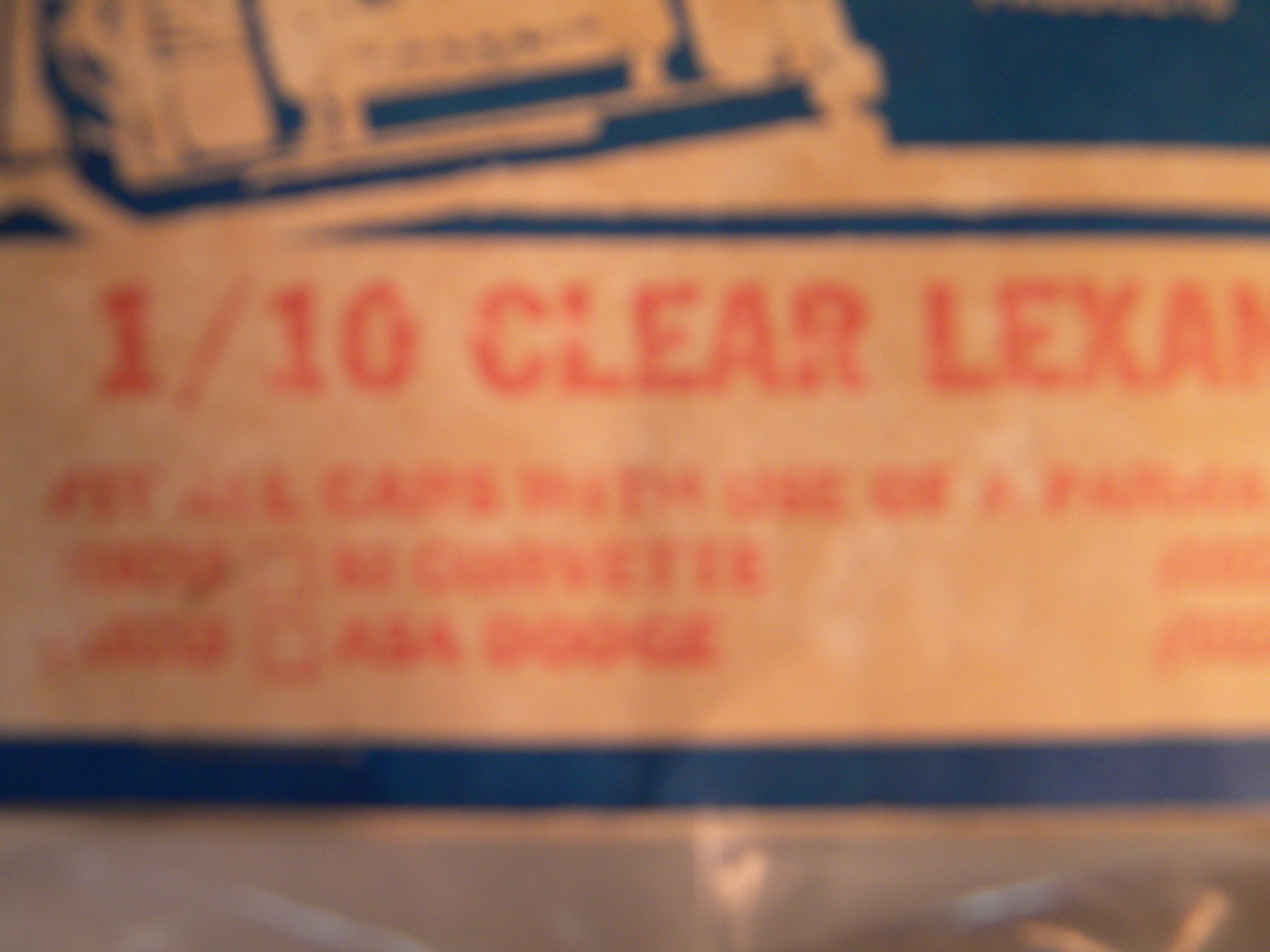This color photograph is an extreme close-up of what appears to be old packaging or labeling, likely from the 1960s. The image is out of focus and blurry, with text in red that is difficult to read clearly. The visible text includes "1/10," "clear," and "L-E-X-A-N," suggesting a product name or specification. The background behind the text is yellowed and discolored, indicating age. Additional words like "CAPS" and "DODGE" can be discerned, hinting that it may pertain to a part or manual related to the Dodge vehicle brand. The lower part of the image features a nondescript gray color, while the top has a horizontal gray line and blue bars at the top and bottom edges. In the upper left corner, there is what seems to be the bottom of a machine before it gets cut off. The right top corner is black. The overall scene is devoid of any people, animals, plants, signs, buildings, or recognizable mechanical objects, focusing solely on the aged and unclear packaging.